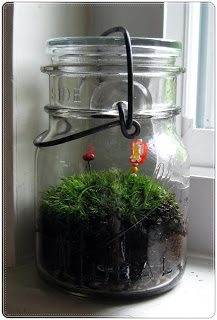The image captures a detailed scene of a small terrarium enclosed in a clear glass mason jar with a vintage, black wire clasp lid. Inside the jar, a verdant mossy plant is thriving, growing halfway up from the soil at the bottom. Embedded within the lush green moss are two decorative red objects that resemble mushrooms, adding a pop of color to the arrangement. The jar is placed on a windowsill in the corner of a room, with a white window frame and light gray walls in the background, creating a minimalist backdrop that accentuates the vibrant plant life within the jar. The windowsill itself is white, and there is a hint of white flooring visible below the frame. The overall effect is a charming juxtaposition of natural and man-made elements within a simple and serene indoor setting.